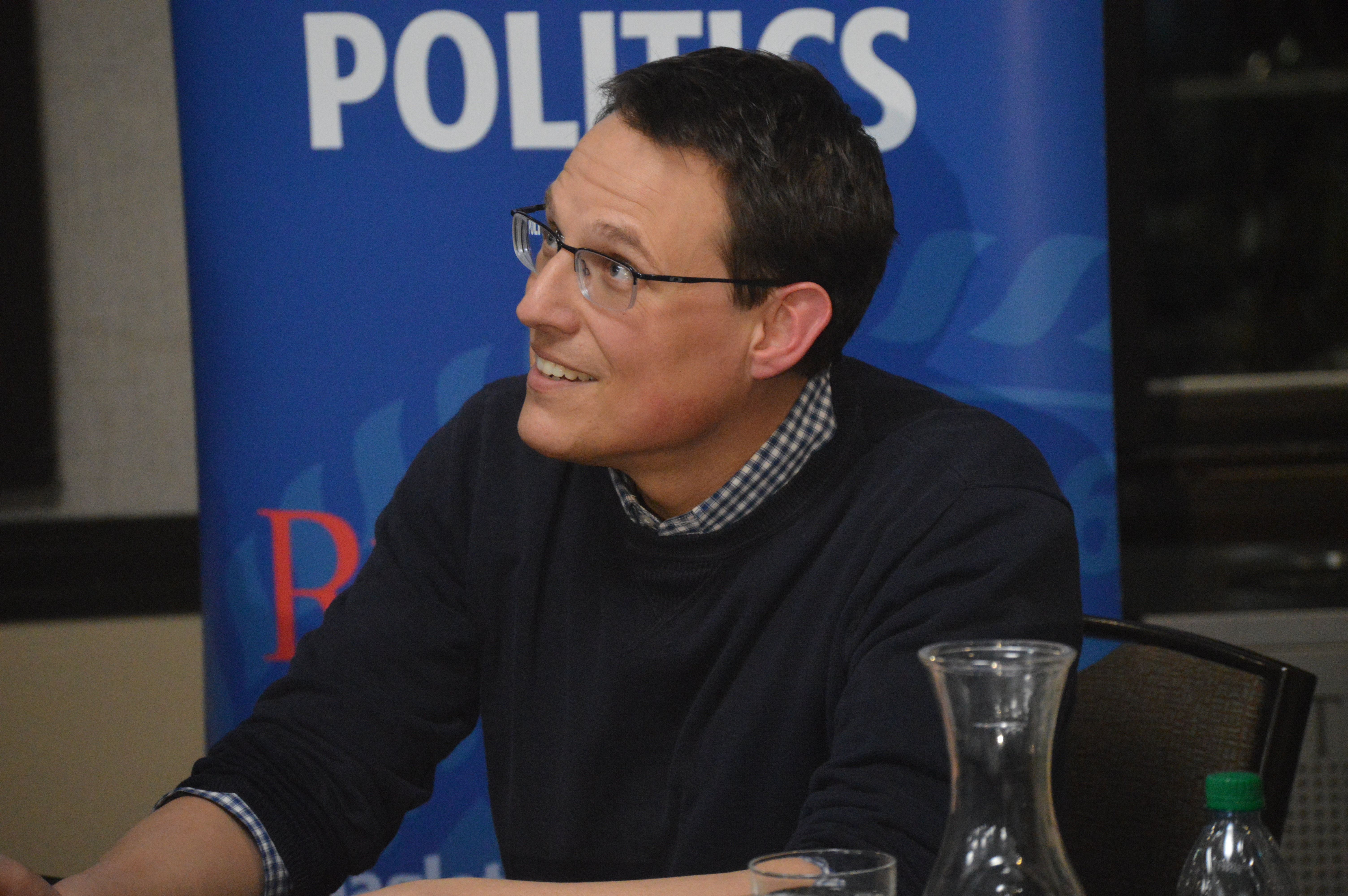The image depicts a bespectacled man with short, dark hair, seated comfortably in a polished, dark-framed chair with a gray cushion. He is smiling and appears engaged in an event, possibly a convention or speaking function, as he looks to his left, seemingly towards someone standing nearby. The man is dressed in a dark-colored sweater layered over a blue-and-white checkered button-up shirt. In front of him, inferred by his posture, is a table laden with a water bottle, a cup, and a vase for drinking, albeit only their tops are visible. Behind him, a blue vertical billboard prominently displays the word "politics" in white, though additional text is obscured by his body. To his right, a piece of furniture or a shelf is partially visible, adding to the setting's detailed ambiance.